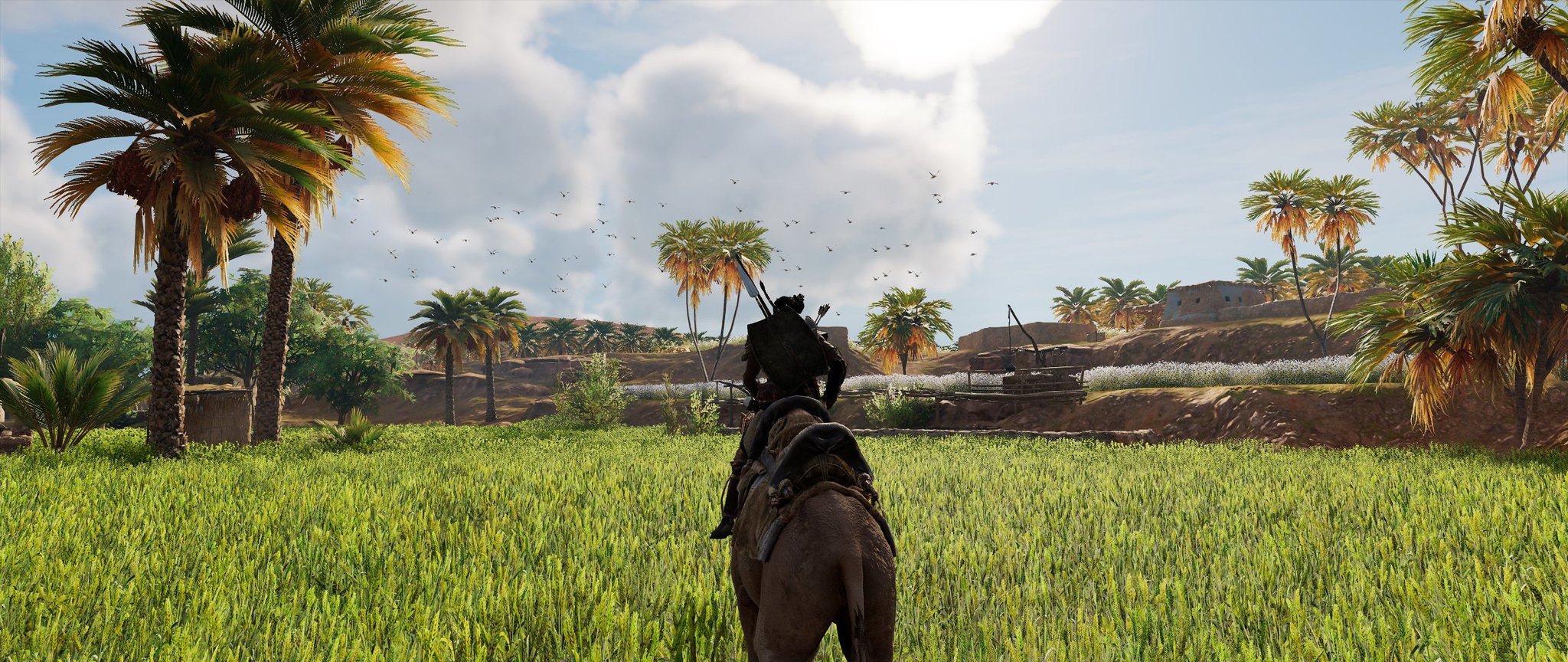This detailed screenshot from a video game captures an expansive landscape viewed from behind, where a silhouetted rider sits atop a brown horse. They are equipped with an assortment of weapons, including a shield, a spear, and a quiver of arrows visibly strapped to their back. The wide landscape format showcases a vast field of tall, green grass stretching out towards gently rolling hills in the background. To the left and right edges of the scene, large palm trees, some bearing substantial fruit, rise above the grass. In the distance, a construction crane-like structure sits atop a slight ridge to the right, blending into the background of scattered buildings and additional trees. The sky is a brilliant blue, dotted with huge white clouds and illuminated by bright sunlight, which casts a natural glow over the entire scene. A flock of birds can be seen soaring through the distant sky, enhancing the sense of a vibrant and animated world.